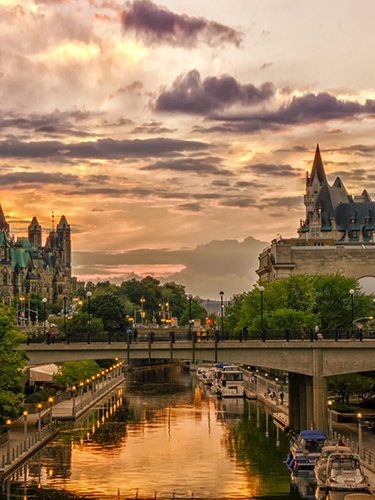This is a detailed vertical photograph capturing a scenic cityscape in Italy. The image centers on a man-made canal flanked by walkways and dotted with boats docked along the right bank. A bridge arches gracefully over the canal, with people strolling across it. Both sides of the canal are lined with evenly spaced streetlights—yellowish on the left and more white on the right—and trees that extend both at the water level and up towards the buildings. 

In the background, a series of tall, cathedral-like buildings—resembling castles with high fort walls—dominate the skyline. The sun is setting, casting a warm golden hue over the scene. Reflections of the sun’s light create a yellowish shimmer on the water’s surface. The sky is a blend of gray, golden, yellow, and orange hues on the left side, with wispy clouds reflecting purples and whites amidst the overcast sky. This picturesque landscape portrays a tranquil river walk, alive with the gentle activity of people and the serene beauty of a European evening.